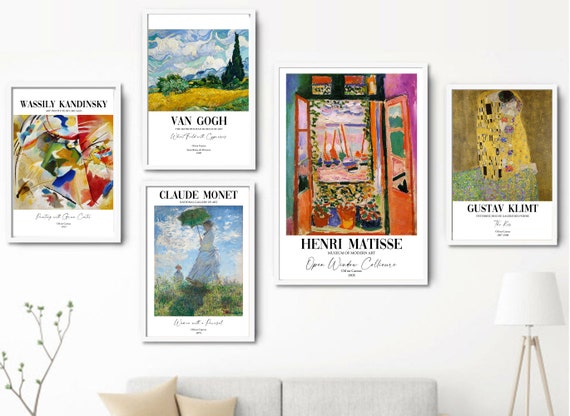This staged photograph features a visually curated gallery wall showcasing five artistic posters, each representing a famous artist and their notable artwork, set within sleek white frames. The arrangement, although appearing edited, conveys a sense of an artful interior space. From left to right, the posters display the works of Wassily Kandinsky, Vincent van Gogh, Claude Monet, Henri Matisse, and Gustav Klimt. The Kandinsky poster highlights a vivid composition with a mix of red, orange, and green. Van Gogh's poster features the iconic "Starry Night" with its swirling blue and white skies. Monet's presents a serene scene of a lady with an umbrella among green grasses. Matisse’s poster captures a lively beach scene with red and blue details. Klimt’s poster details an intricate and colorful depiction, possibly "The Kiss," with rich golds and blues.

Beneath this art display, you can see the top of a modern, two-seat gray fabric couch adorned with two tan-colored cushions. To the left, a brown stick with green foliage brings a touch of nature, while to the right, a stylish floor lamp with three legs and a white lampshade adds elegance to the scene. The interplay of shadows and textures hints at a digital alteration, enhancing the images' placement on the pristine white wall.